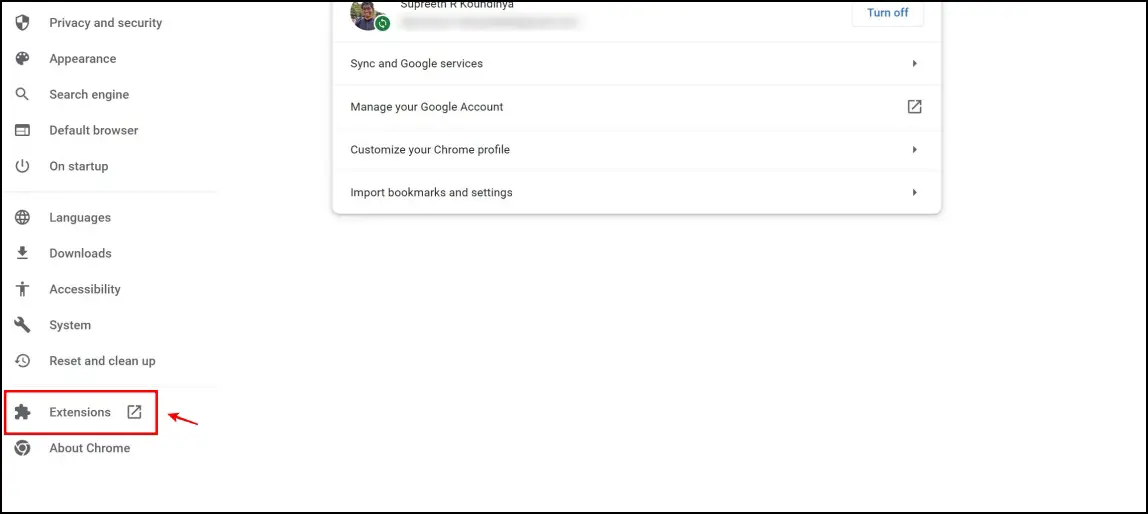The image displays a user interface menu on a white background, presumably from a Google Chrome settings page. On the left-hand side, there is a vertical list of settings categories, including "Privacy and Security," "Appearance," "Search Engine," "Default Browser," "On Startup," "Languages," "Downloads," "Accessibility," "System," "Reset and Cleanup," "Extensions," and "About Chrome." A red rectangle highlights the "Extensions" category, with a red arrow pointing towards it, drawing attention to this section.

In the central part of the image, a dropdown menu showcases several options: "Sync and Google Services," "Manage Your Google Account," "Customize Your Chrome Profile," and "Import Bookmarks and Settings." In the top-right corner, there is a white button labeled "Turn Off."

Adjacent to the button, a profile picture of an Indian man is displayed. This individual has dark hair, dark skin, and is wearing a blue shirt. Though the name is partially cut off, it appears to read "Supreetnrk Kounainya" or a similar variation. Additionally, there is a green circular icon with arrows forming a loop near his profile picture, likely indicating an active sync status.